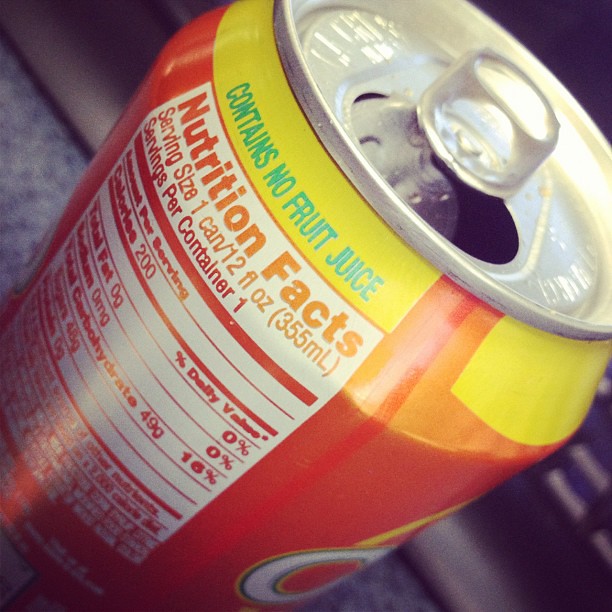The image is a close-up, color photograph of an open aluminum can of juice taken from a slightly elevated angle, showing the top half of the can tilted diagonally towards the bottom left corner. The can's design features a prominent yellow banner at the top with the blue text "contains no fruit juice." Below this banner are the nutritional facts, which indicate one serving per container of 12 ounces, 200 calories, 0 grams of total fat, 0 milligrams of sodium, and 49 grams of total carbohydrates. The majority of the can's body is a light red-orange color, and it rests on a gray surface speckled with blue. Drops of liquid are visible on the opened lid, suggesting it may be empty. Part of a logo or brand name is partially visible near the bottom right but is indiscernible.